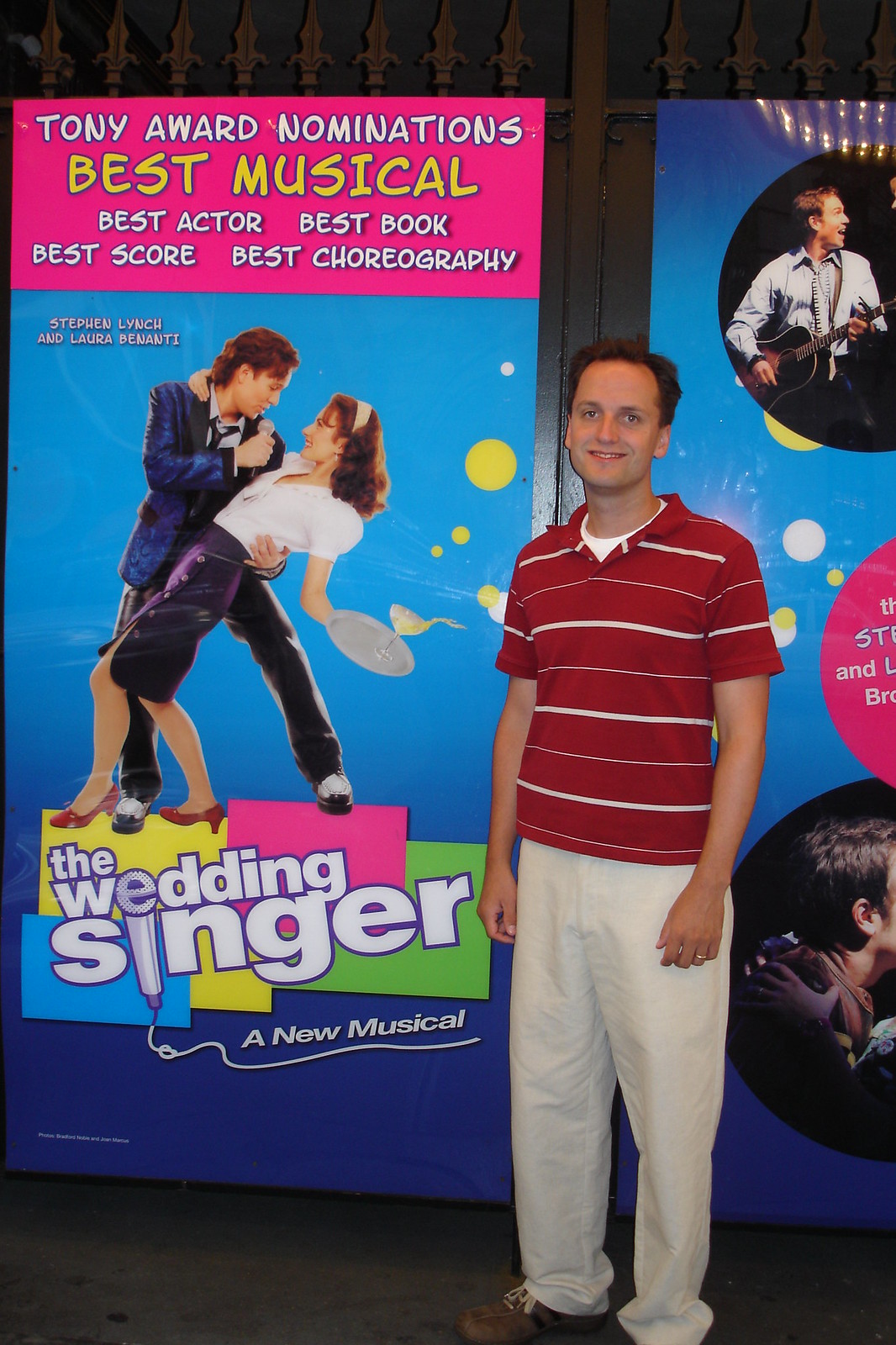The image shows a man with short black hair, wearing a red polo shirt with horizontal white stripes in a pattern of thicker and thinner lines, and white pants. His hands rest by his sides, fingers slightly curled, and he is smiling with his teeth visible. Behind him, there are two long posters, predominantly blue with a pink top section. The poster to the left, which is more visible, displays white and yellow text that reads, "Tony Award Nominations: Best Musical (in yellow), Best Actor, Best Book, Best Score, Best Choreography." Below this, it lists "Stephen Lynch and Laura Benanti" and features an image of the two actors in a dramatic pose: Lynch serenading Benanti, who is dressed as a waitress, bending backward while holding a tray with a tipping drink. At the bottom of the poster is the logo for "The Wedding Singer, A New Musical," where the 'E' and 'I' in "Wedding" and "Singer" combine to form a microphone. The man stands just right of center, part of his black shoes partially cut out of frame.